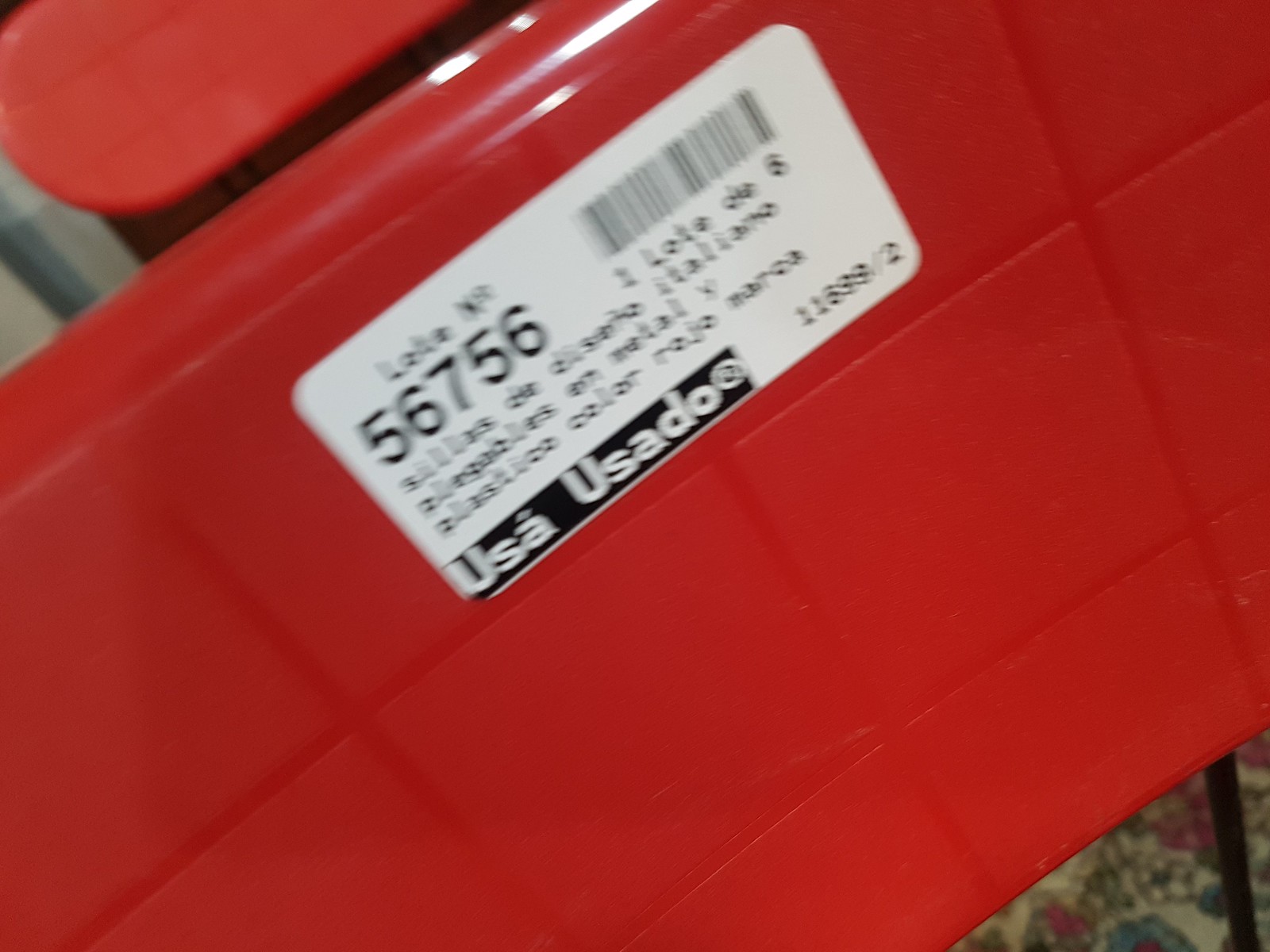This is a close-up photograph of a bright red, textured surface, potentially made of plastic or metal, which resembles a tabletop or the back of a chair. The surface is divided into several visible square tiles. In the bottom right corner, there is a glimpse of a carpet with a floral pattern in cream, red, and blue, outlined in black, along with a black metal pole intersecting the scene. Affixed to the red surface is a slightly blurry white, rectangular sticker with rounded edges. This sticker features black text and numbers, prominently displaying "56756" on the left and a barcode on the right. Below the barcode, there are additional letters and numbers which are too out of focus to decipher clearly. In the lower left of the sticker, within a black box, the white letters "USA" and "USA DO" are distinctly visible. Additionally, there is a sequence in black print reading "11699/2" off to the side.